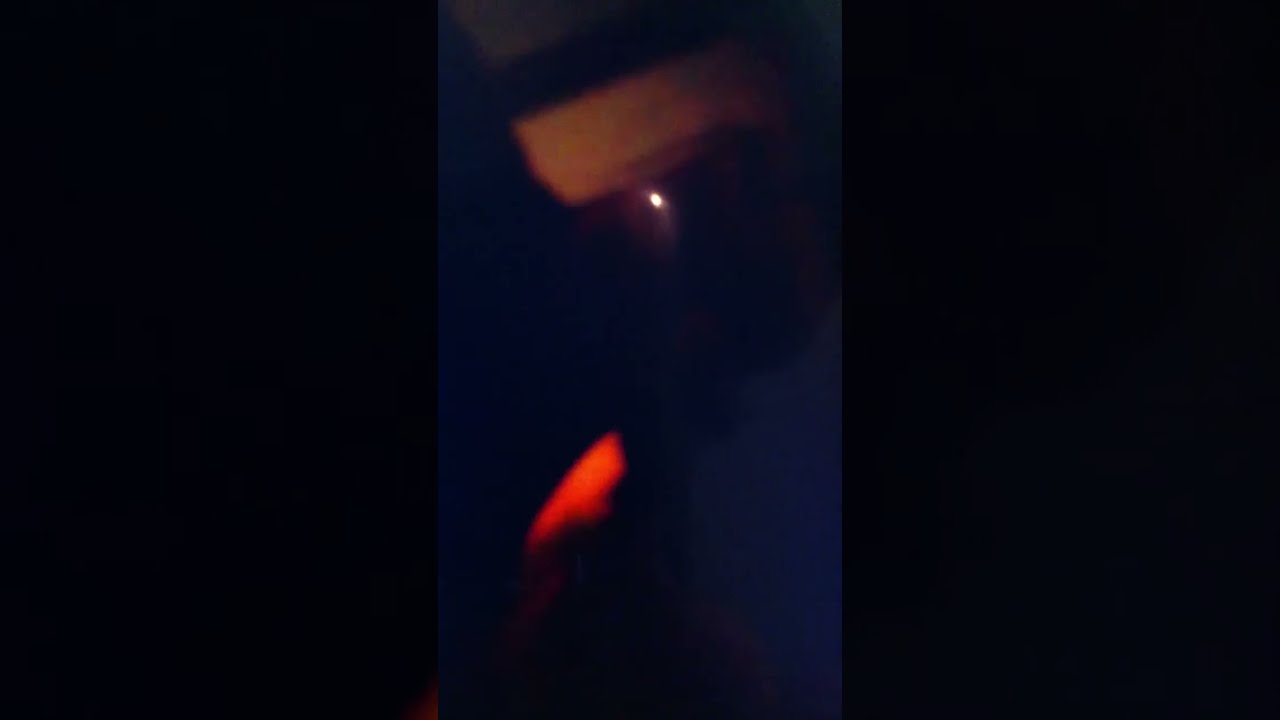This is a very dark photograph, predominantly black with certain variations in tone. The image appears to be divided into three vertical panels: the left and right panels are solid black, while the middle panel is a very dark blue, suggesting a midnight sky. In the top section of the middle panel, there is a small, round, orange-yellow glowing orb. This light source, potentially the moon, a distant aircraft, or a tower beacon, stands out against the uniformly dark background. The region surrounding the light has a circular area of slightly lighter dark blue, perhaps due to atmospheric fog or clouds, enhancing the glow and adding a mysterious quality to the scene. The overall effect is a striking contrast between the intense darkness and the solitary, enigmatic light.